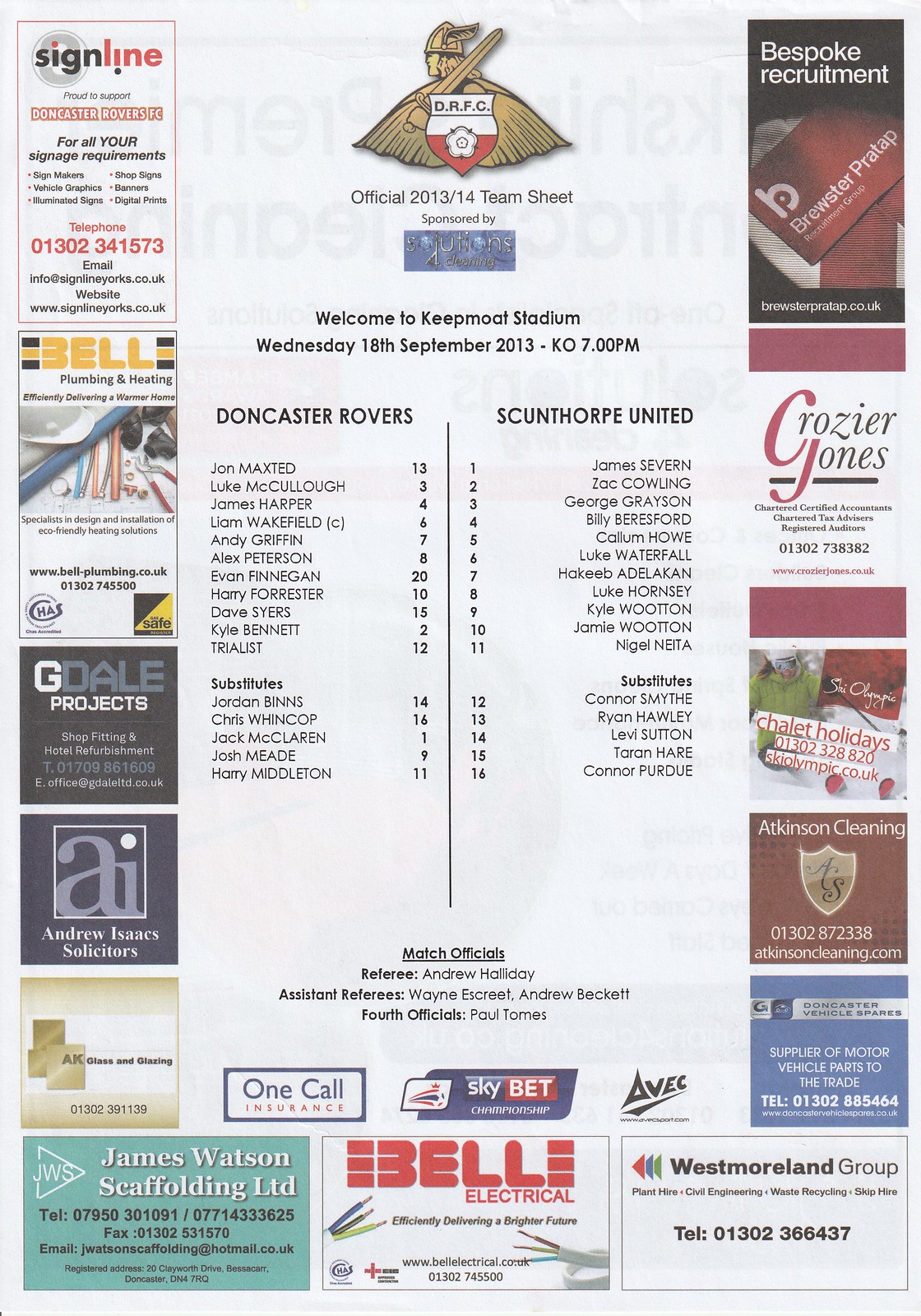This image is an official 2013-14 team sheet for a soccer match between Doncaster Rovers and Scunthorpe United, held at Keepmoat Stadium on Wednesday, 18th of September 2013, with a kickoff at 7 p.m. The document features a central multi-color print with a Viking symbol and "DRFC" on a shield. It lists the players for both teams: Doncaster Rovers' starting lineup includes John Maxted, Luke McCullough, James Harper, Liam Wakefield, Andy Griffin, Alex Peterson, Evan Finnegan, Harry Forrester, Dave Syers, Kyle Bennett, and a trialist, with substitutes Jordan Binns, Chris Whincop, Jack McLaren, Josh Meade, and Harry Middleton. Scunthorpe United's lineup comprises James Severn, Jack Cowling, George Grayson, Billy Brashford, Callum Howe, Luke Waterfall, Keevyn Arlaud, Levi Sutton, Jamie Wootton, Nigel Neita, and substitutes Connor Smith, Ryan Hawley, Levi Sutton, Tom Pugh, and Kyle Wootton. Match officials for the game include referee Andrew Haines, assistant referees Wayne Grunnill and Andrew Beckett, and fourth official Paul Thompson.

The sheet also includes numerous advertisements from sponsors such as One Call Insurance, G. Dale Projects, Andrew Isaacs Solicitors, AK Glass and Glazing, James Watson Scaffolding, Bell Electrical, Sky Bet Championship, ABEC, Westmoreland Group, Doncaster Vehicle Spares, Atkinson Cleaning, Chalet Holidays from the Sky Olympic, Grozier Jones, and Bespoke Recruitment, displayed along the left, bottom, and right sides of the document. The venue warmly welcomes attendees to Keepmoat Stadium for this event.